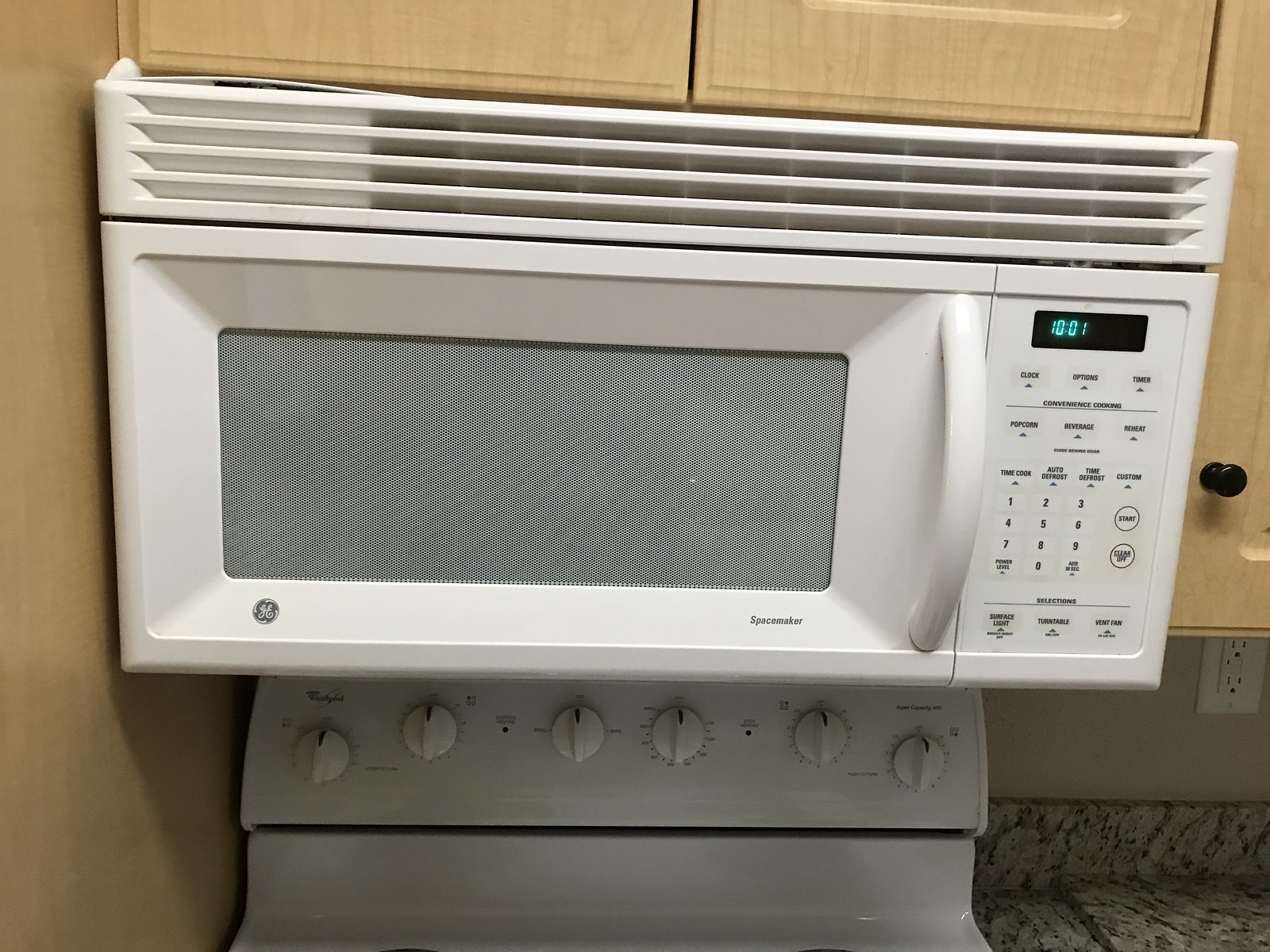The photograph captures a kitchen scene featuring a General Electric Spacemaker microwave oven with a white door and face, prominently displaying a green digital clock set to 10:01. The microwave is installed beneath light-colored wooden cabinets with black handles and has a vent at the top. Situated directly below the microwave is the top part of a white stove with six dials visible, but the burners remain out of sight. To the right of the stovetop, in the bottom corner of the image, lies a granite countertop speckled with shades of gray. An electrical outlet is mounted on the lightly colored wall above the countertop, and the overall focus of the image is on the microwave and its integration into the kitchen setup.